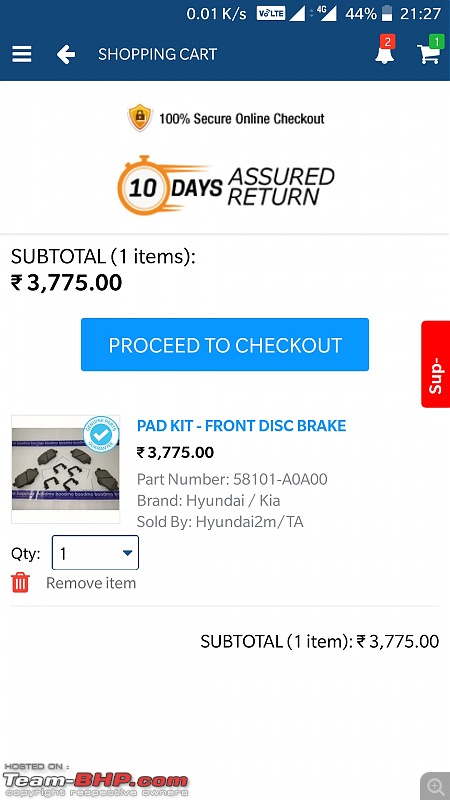This screenshot from a mobile app displays an online shopping interface. At the very top, there is a blue banner that includes mobile status icons, with the time showing 21:27, a battery icon indicating 44% charge, and a hamburger menu icon. A left arrow for navigating back to the previous screen is placed next to the title "Shopping Cart." On the right side of the banner, there is a notification bell with a red badge displaying the number 2 and a shopping cart icon with a green badge displaying the number 1.

Below this banner, the white background of the main content area highlights several important details. Firstly, logos indicating "100% Secure Online Checkout" and "10 Days Assured Return" are prominently displayed. The subtitle "(1 item)" follows, noting a single item costing €3,775. A blue "Check Out" button is positioned underneath.

The product being purchased is depicted with a photo of the item, identified as a "Pad Kit Front Disc Brake" including the part number. It is specified for Hyundai or Kia vehicles, with a quantity of 1. The subtotal for this purchase is clearly listed as €3,775.